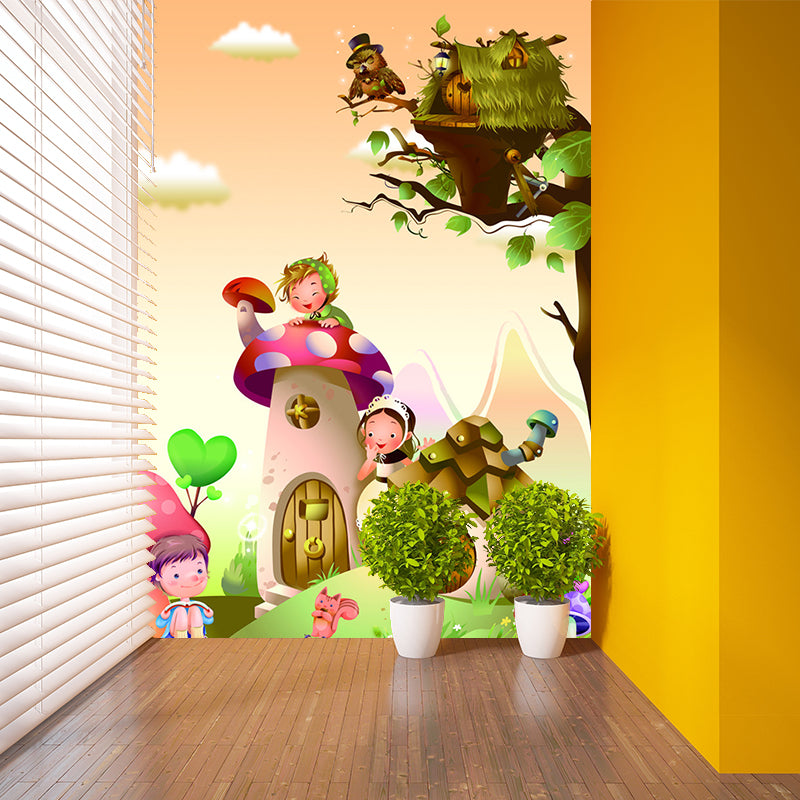The image depicts a whimsical children's mural on a wall, set in a brightly lit room with various elements creating a playful and vivid scene. The right wall of the room is painted mustard yellow, while the left features floor-to-ceiling white Venetian blinds partially opened to allow sunlight in. The floor is made of polished, rustic hardwood.

Central to the image is the mural, characterized by its colorful and animated design, likely intended for a child's playroom. The mural showcases an imaginative scene with two large mushroom houses. One mushroom features a tan base and a red, polka-dotted cap, with a doorway and window. Perched atop this mushroom is a cartoon child with brown hair, dressed in a green outfit and headband. Adjacent to it, another mushroom house, also vividly red, has a smaller attached mushroom serving as a chimney.

On the mural’s right side, there's a treehouse nestled within a tree, topped with a thatched grass roof. An animated owl wearing a top hat sits beside a small, heart-shaped door. Below, a girl dressed in a maid-like black and white outfit stands at the base of the mushroom, while a small boy sits cross-legged on the ground reading a book, surrounded by a pink squirrel and vegetation with heart-shaped leaves.

The foreground of the photo features two identical white pots with perfectly round, green bushes, which appear to be digitally replicated, adding a touch of modernity to the enchanted scene. The mural's backdrop includes a serene, pastel mustard sky with fluffy clouds, adding to the overall charm and fantasy of the setting.